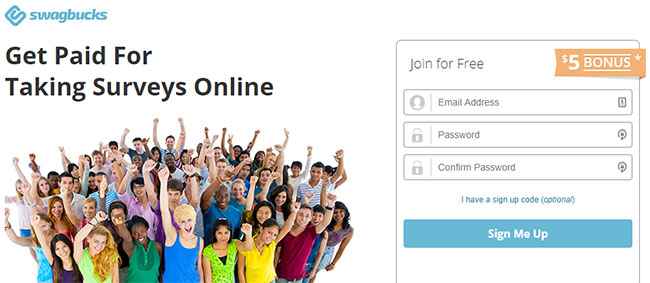The image depicts the homepage of the Swagbucks website. In the top left-hand corner, the word "swagbucks" is displayed in lowercase letters in blue font, accompanied by a small blue icon. Directly below, in larger, bold black letters, the website promotes earning money by taking online surveys with the text: "Get paid for taking surveys online."

The central part of the image features a cheerful, large group of people with their arms raised, appearing to be shouting and smiling, symbolizing excitement and satisfaction. Adjacent to this group, a bordered sign-up section invites users to "Join for free," followed by an orange text box with white text offering a "$5 bonus."

Below this prompt, there are fields to input personal information: "Email address," "Password," and "Confirm password." Additionally, a small blue text link indicates an optional field for a sign-up code: "I have a sign-up code (optional)."

At the very bottom of the right-hand side, a blue-bordered text box includes a sign-up button in blue with white, partially capitalized text reading "Sign Me Up," with the letters S, M, and U in uppercase. Overall, the image presents a call-to-action inviting users to register and start participating on the Swagbucks platform.